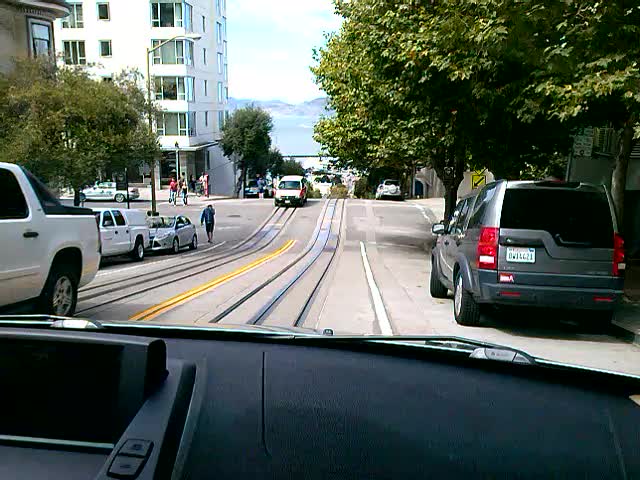A scenic photograph taken from the passenger seat of a car in San Francisco, California. The image captures the view through the windshield, with the car's black dashboard visible at the bottom of the frame. The roadway ahead, seen from the passenger side, features dark train trolley tracks running centrally from the dashboard towards the horizon. The road is marked with a double yellow line, indicative of a two-way street. 

To the immediate right, a car is parked underneath a lush, bushy tree, while the left-hand lane is occupied by several cars, both parked and moving. The vehicle appears to be descending a steep hill, and the gradient of the road reinforces San Francisco's famously hilly landscape. 

In the distant background, a series of mountains and a body of water are visible, adding depth and context to the urban scene. To the left side of the road, tall trees and a high-rise residential building create a vertical balance, while a cross street intersects the main road at a four-point intersection that the car is approaching. The blend of natural and man-made elements, along with the dynamic perspective of the downhill journey, captures the unique essence of San Francisco's cityscape.